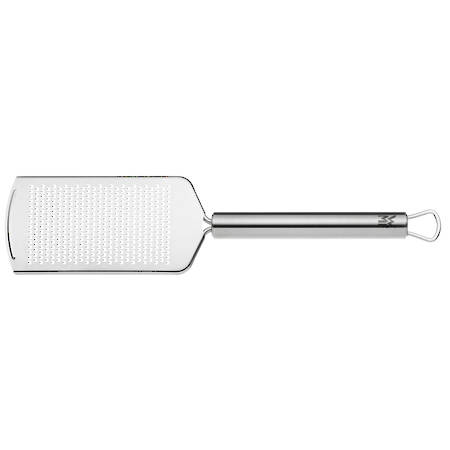The image depicts a silver handheld grater with a long, round handle, placed horizontally on a completely white background. The grater features a wide, flat paddle-like body with numerous small holes for fine grating, suitable for tasks like grating garlic or ginger. The tool is meticulously detailed: the grating surface is positioned on the left, and the smooth, stainless steel handle extends to the right. An engraved marking—showing a capital W above a capital M—adorns the very bottom of the handle. Additionally, a steel hook is integrated into the handle, allowing for easy hanging. The edges of the paddle have a thick metal border, and a subtle black edging runs along the outside. The grater's sleek design and practical features make it a versatile utensil for any kitchen.